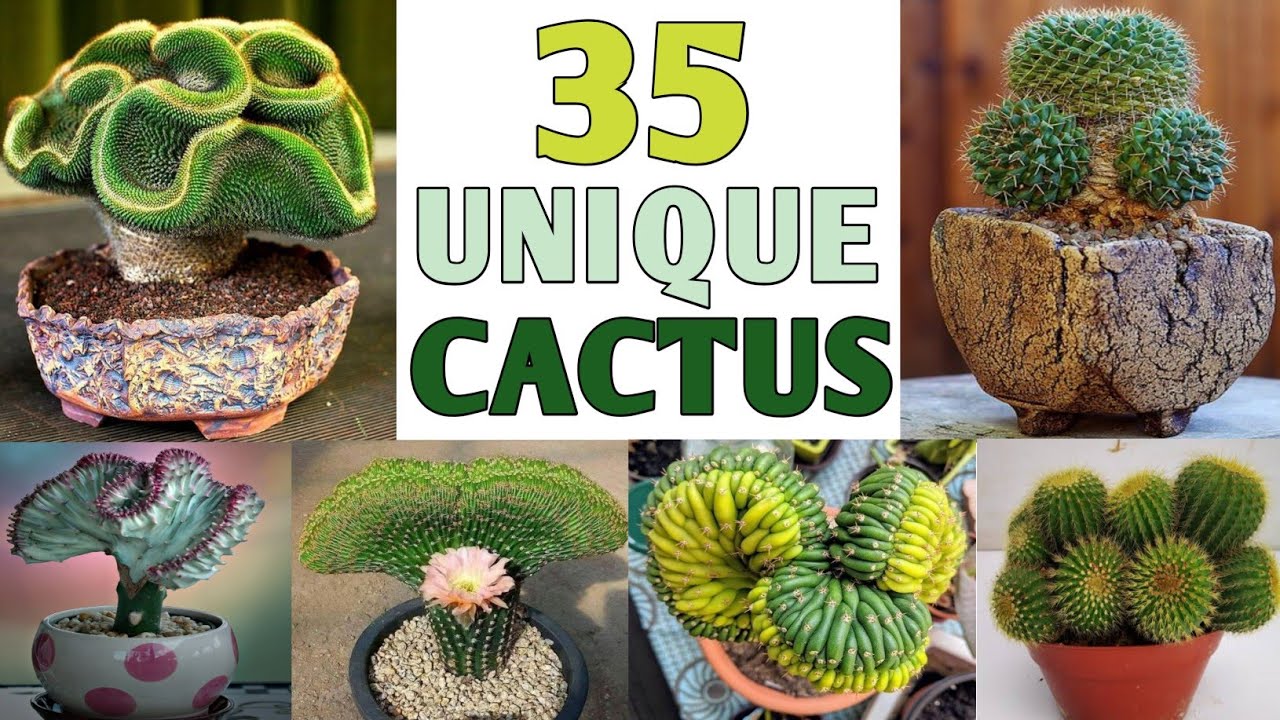The image titled "35 Unique Cactus" prominently displays text in three different shades of green: a light pea green, a pale green, and a forest green. This text is centered at the top of the image. Surrounding the text are six unique photographs of various cacti, arranged in a grid with three images on the top and four on the bottom.

On the upper left, there is a cactus with numerous folds curling inwards, housed in a dented, multicolored stone pot with hues of blue, yellow, and orange. To its right is a cactus with spherical, spiny protrusions emerging from an earthy pot that appears uprooted but is likely designed that way. In the upper center, above the grid, the title "35 Unique Cactus" is displayed in distinct shades of green.

Below, on the lower left, there's a light green cactus with purple-edged folds and a dark green stem, placed in a white, egg-shaped pot adorned with pink dots. Next to it is a cactus featuring a cylindrical base and a fan-like top resembling a fishtail, crowned with a pink flower and yellow center, set in a black pot filled with rocks.

Further right, there's a cactus with bean-like segments in varying shades of green, set in a clay pot alongside assorted items, including a blue and gray striped object. Finally, the bottom right showcases several rounded cacti clustered together in a red pot.

Each of these visually unique cacti is displayed in individual pots, emphasizing distinct textures and colors, making the entire composition rich in detail and diversity. This image resembles a header for an article or a poster, designed to intrigue viewers with its array of unusual and aesthetically striking cacti.